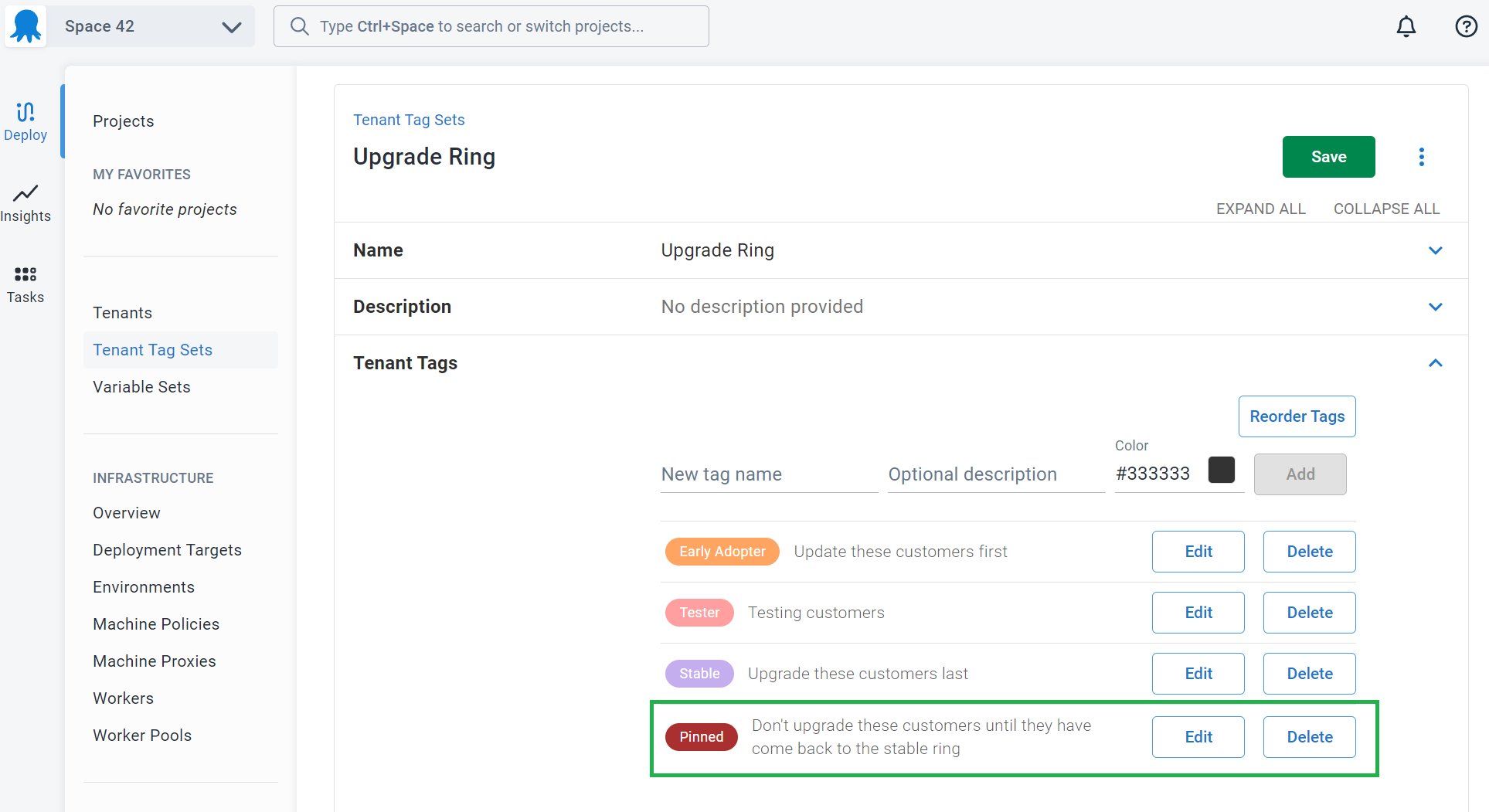**Detailed Image Description:**

The image is a computer screenshot displaying a web-based management dashboard. The top navigation bar is predominantly black with a blue section. In the upper-left corner, the word "default" is visible, and in the upper-right corner, it says "library." The navigation bar features several menu options: "Dashboard," "Projects," "Infrastructure," "Tenants," "Library," "Tasks," and "Configuration," as well as a search bar and an "Administrator" label. The word "Library" is highlighted in a darker shade, indicating it is the currently selected section.

Under the "default" label, "Library" is mentioned again, reinforcing the current active section of the dashboard. Dominating the center of the image is a large white rectangular area, titled "Tenant Tag Sets - Upgrade Ring." Below this title, there are two columns labeled "Name" and "Description."

The first row under these columns reads:
- **Name:** Upgrade Ring
- **Description:** Describes which upgrade ring the tenant belongs to.

The first item within this section is an oval with a yellow background labeled "Early Adopter," accompanied by the description "Update these customers first." Next to this oval are blue "Edit" and "Delete" buttons.

The second item features a green oval labeled "Stable," with the description "Upgrade these customers last." It is also accompanied by blue "Edit" and "Delete" buttons.

Towards the bottom of the white rectangle, there is a large, green-circled section marked in red with a label "Pinned." It instructs, "Don't upgrade these customers until they have come back to the stable ring." This section also includes blue "Edit" and "Delete" buttons.

Overall, the screenshot captures the detailed configuration settings for managing tenant upgrade rings within the library section of a dashboard.